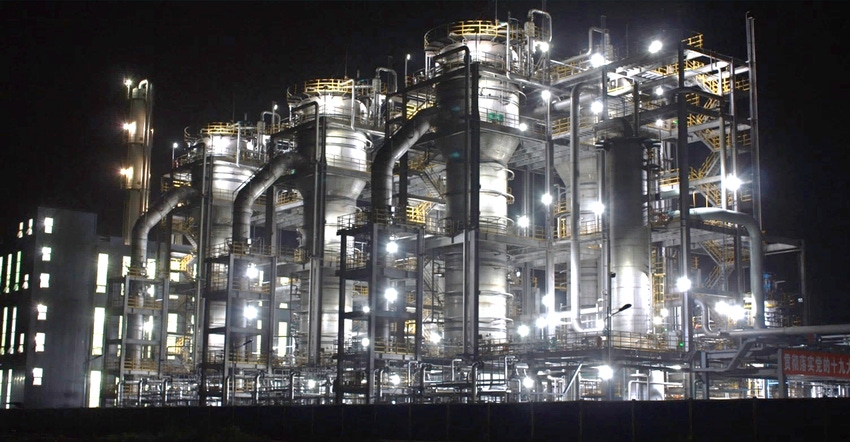This night-time image is a detailed 3D color rendering of a brightly lit fuel production facility set against a pitch-black sky and a black strip border at the bottom. The facility, occupying most of the frame, features a series of towering, white cylindrical structures that taper downwards, capped with flat platforms enclosed by fencing rails. These towers are encased in open-air vertical rectangular girder frameworks, with a series of flights of stairs providing access to different levels. On the left side are two rows of three such towers, framed one behind the other. Adjacent to these towers is a substantial gray block building, approximately three stories tall, adorned with large windows on each level. The entire scene is illuminated by numerous floodlights, highlighting the intricate network of pipes and chutes that interlace through the facility, enhancing the industrial aesthetic of the rendering.